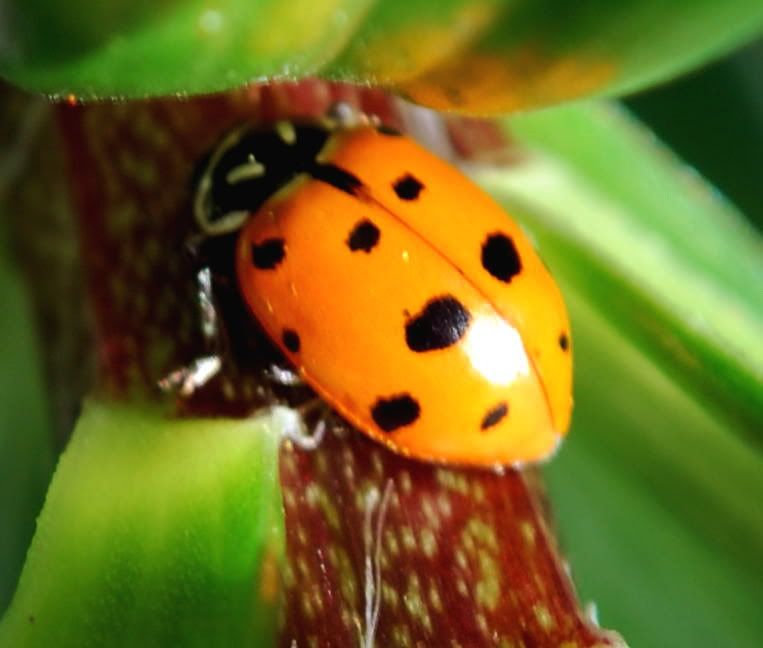This detailed, square-shaped image features an extreme close-up of a ladybug perched on a plant. The ladybug, occupying the center of the frame, has a light orange shell adorned with black spots, and a distinctive light reflection creating a shiny spot on its back. Its black head, outlined in white with two white dashes resembling eyes, is angled towards the upper left corner of the photo, while its slightly blurred body faces the bottom right. The plant it is on has a prominent red part speckled with yellow dots, contrasting the large, glossy green leaves around it. The leaves, some curling off the edge of the frame, reflect the light, with an orange tinged reflection likely from the ladybug shell itself. Overall, the left side of the image transitions into darkness, adding depth and contrast to this natural and potentially backyard setting.